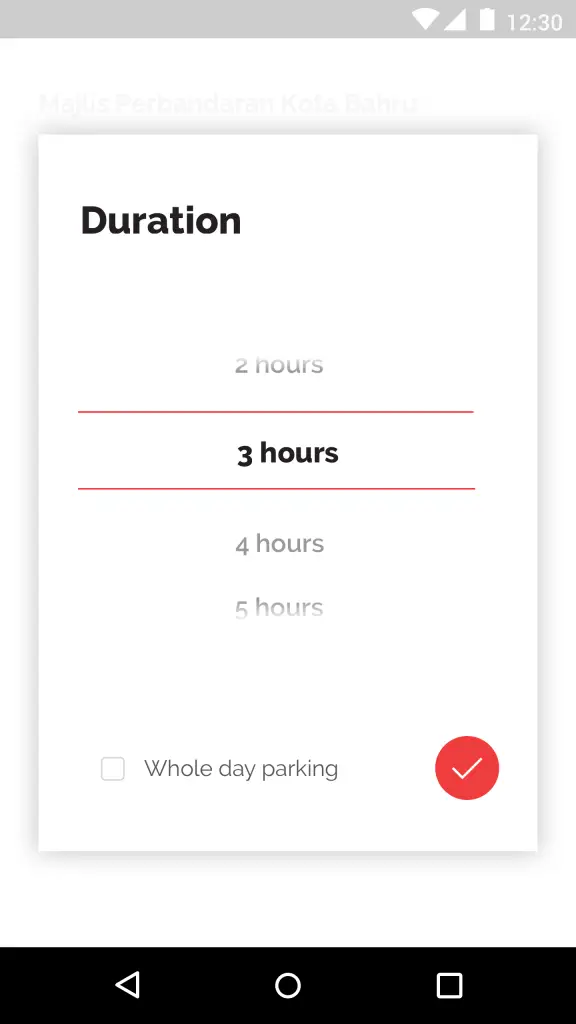A cell phone screenshot displays a duration selection page. At the top right corner, a thin gray bar stretches across the screen housing several icons in white: a Wi-Fi icon, a cell phone reception icon, a battery icon, and the time, which reads 12:30. 

Below this bar, set against a white background, is a white pop-up box with subtly shadowed edges enhancing its pop-up effect. Positioned two spaces down and one space to the right within the box is the text "DURATION" in black, bold capital letters. Presented below are scrollable duration options, with the selection currently set to three hours.